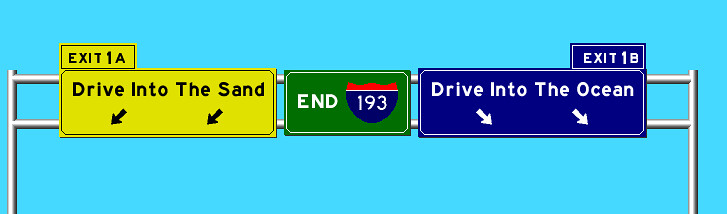This is a digital rendering of an overhead highway sign arrangement against a light blue background, featuring three distinct signs mounted on silver metal poles. On the far left, there is a yellow rectangular sign with black text that reads, "Exit 1A, drive into the sand," accompanied by two black arrows pointing left. The central sign is green and rectangular, displaying the message "End of route 193" in white letters, indicative of a highway termination point. On the far right, a blue rectangular sign with white text humorously advises, "Drive into the ocean, exit 1B," with two white arrows pointing downward to the right. The signs and their improbable instructions suggest a whimsical, computer-generated image rather than a realistic road guide.